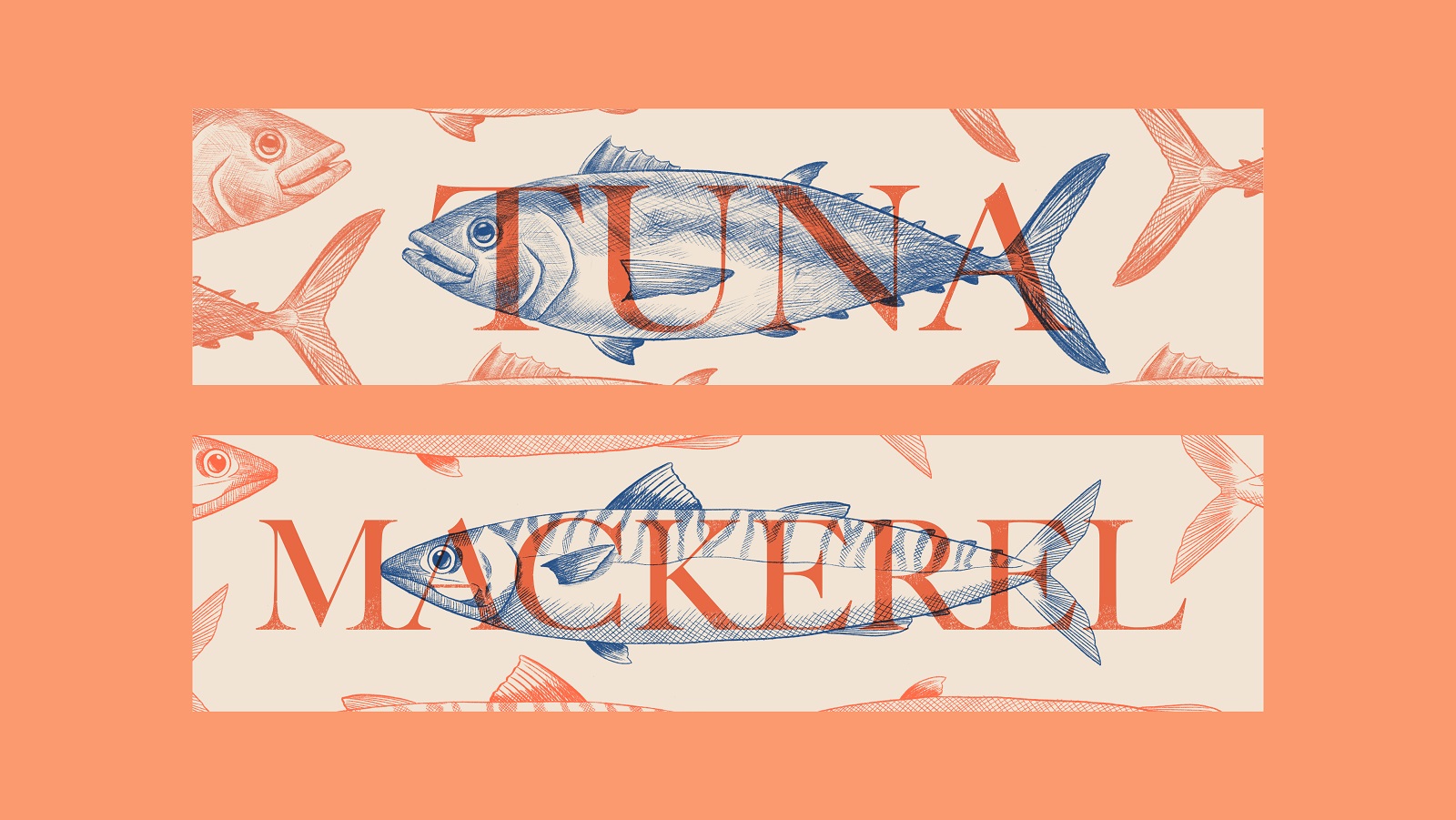The image features two distinct rectangular drawings of fish, each bordered by a large orange frame that divides them. The top rectangle depicts a blue tuna fish with an almond-shaped body and a large tail, imposed over a tan background. The word "TUNA" is written in bold orange text above the fish. Additional tails and a single head of a tuna are placed along the outer border of the top rectangle. On the bottom, the image showcases a longer, more oval-shaped mackerel fish with pointed ends, two dorsal fins, fins on its stomach, and two tail fins, also set against a tan background. The word "MACKEREL" is displayed in orange text above this fish. The heads of both fish are oriented toward the left side of the picture while their tails point to the right. The overall background of the image has a light orangey or pinkish shade.